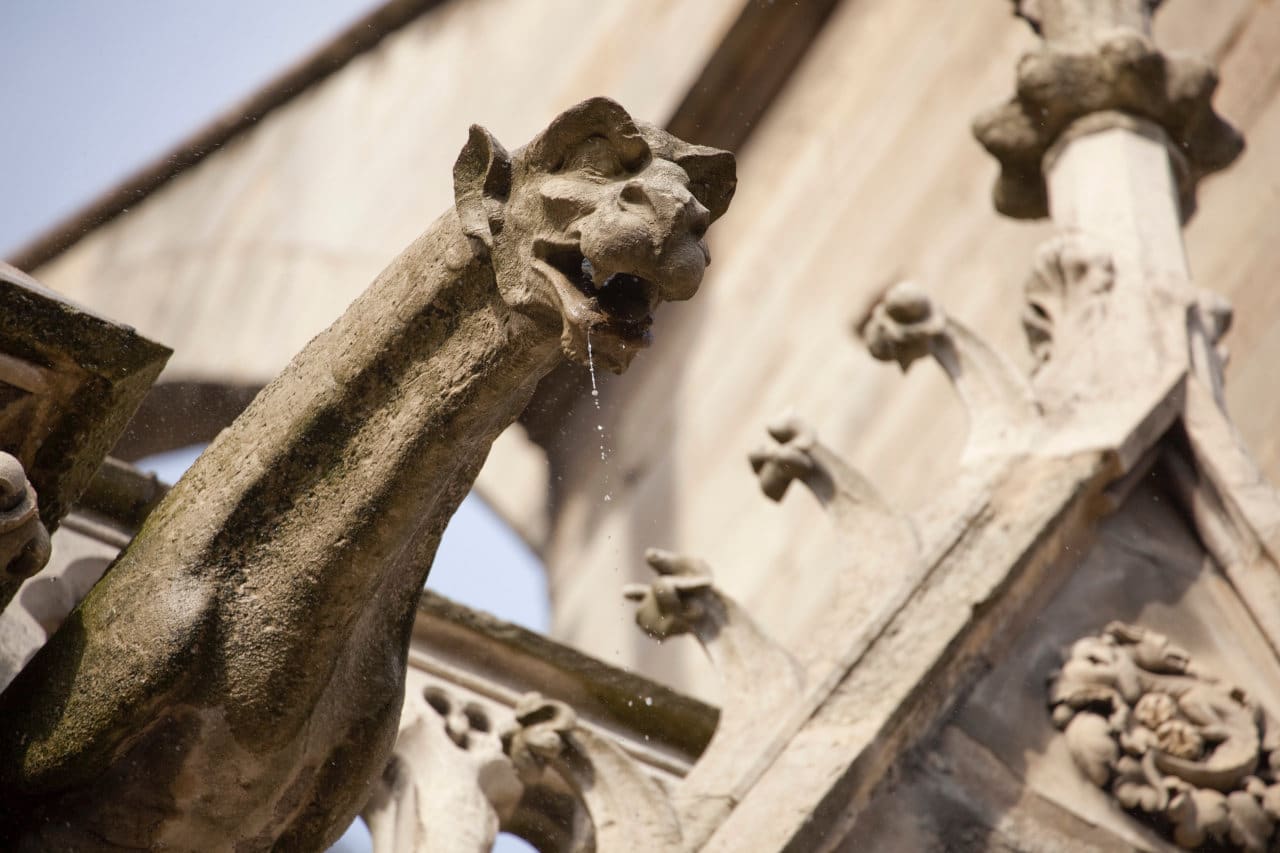The photograph captures the side of a cream-colored, ornate building, possibly a church or heritage monument, taken from a low angle. The main focus is a detailed gargoyle situated prominently in the middle of the scene, appearing just below the camera, with deep hooded eyes, pointed ears, and a monstrous, fantasy-era face. The gargoyle, covered in brownish-black hues and metallic textures, has its mouth open, from which water seems to be dripping, adding a lifelike and eerie touch as though it had just rained. Surrounding the gargoyle, the building's exterior is adorned with intricate designs, including what look like creepy hand-like protrusions and an ornate fleur-de-lis near the peak of the building's architecture. In the background, against a backdrop of white and beige, the blue sky peeks through, adding to the grandiosity of the scene. A railing runs behind the gargoyle, integrating seamlessly with the elaborate stonework and further enhancing the image's architectural splendor.